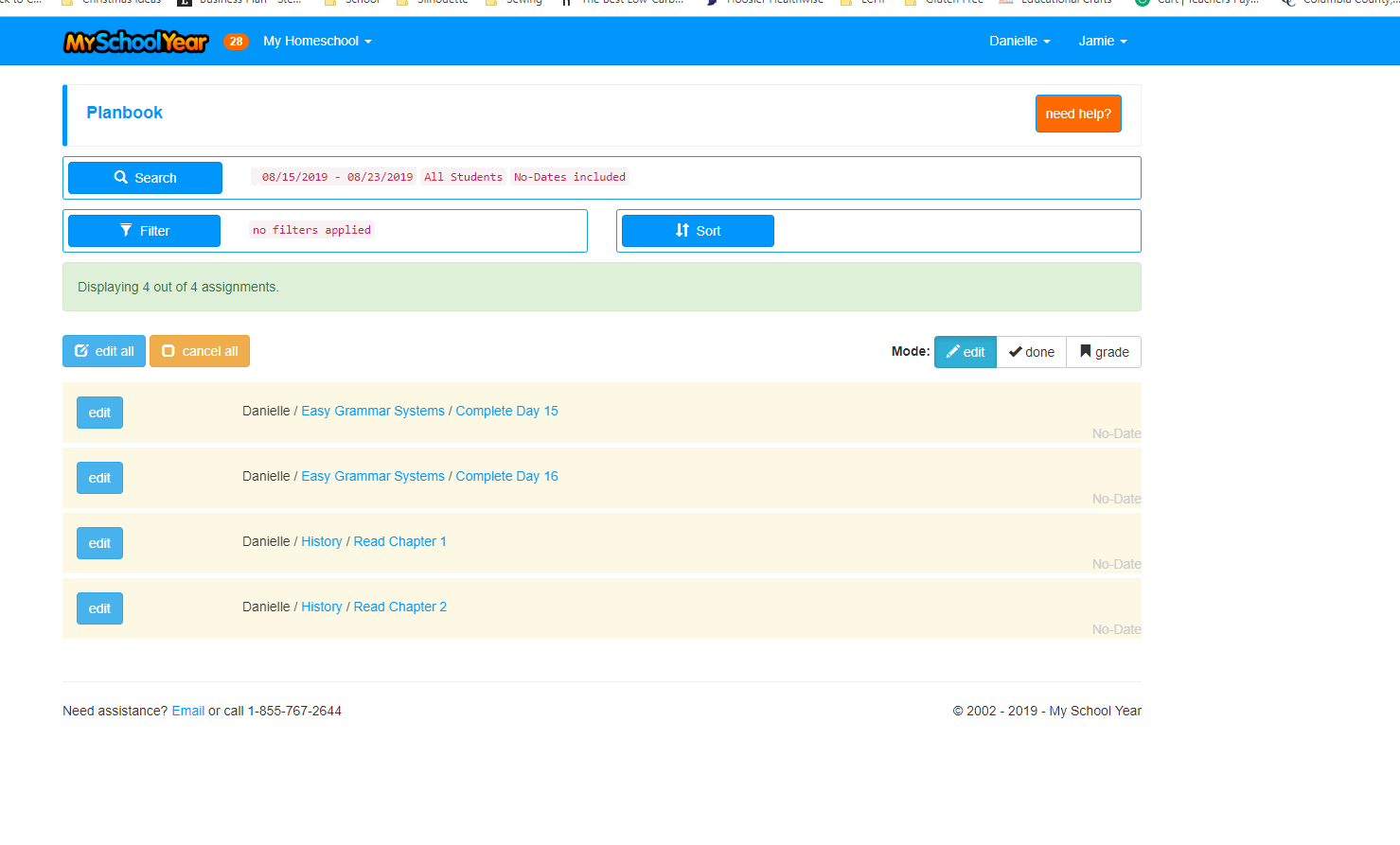**Detailed Caption:**

The image displays a webpage from the site "My School Year," tailored for homeschooling. At the top left, the title "My Home School" appears alongside the number 28. On the top right of the page, there are two names, "Danielle" and "Jamie," each with accompanying drop-down menus. The main section is labeled "Plan Book" and is set to show all students with a weekly view.

A "Need Help" button is available for assistance, and options for "Filter" (no filters applied), "Edit All," and "Cancel All" are present. Under Danielle's schedule, the entries include "Easy Grammar Systems, complete day 15" followed by "Easy Grammar Systems, complete day 16." Additionally, there are history assignments: "Danielle History, read chapter one" and "Danielle History, read chapter two."

The interface is currently in edit mode, with buttons for "Done" and "Grade" visible. The layout appears straightforward, aimed at allowing homeschoolers to organize and manage their lessons efficiently, providing a structured approach akin to a traditional school environment. The overall design is simple and user-friendly.